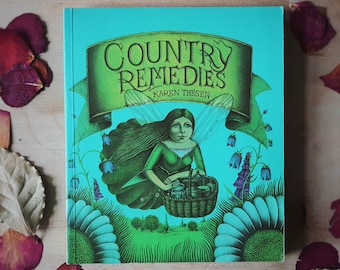The image shows the front cover of a book titled *Country Remedies,* authored by Karen Thyssen. The book, which appears to be a hardback, is placed on a wooden table with a scatter of predominantly red flower petals and a few white ones surrounding it. The cover features a subdued color palette and an illustration of a female fairy with long dark hair, donned in a flowing green gown, and clear wings extending from her back. The fairy gracefully flies over a meadow-like field, carrying a basket on her arm. She is flanked by two purple flowers with weeping bell petals located at the bottom corners of the cover. The background transitions from a light blue sky to grassy terrain. The title *Country Remedies* is displayed on a banner, adding to the old-world charm of the cover art. The image presents a quaint and whimsical scene, rich in detail and illustrative finesse.